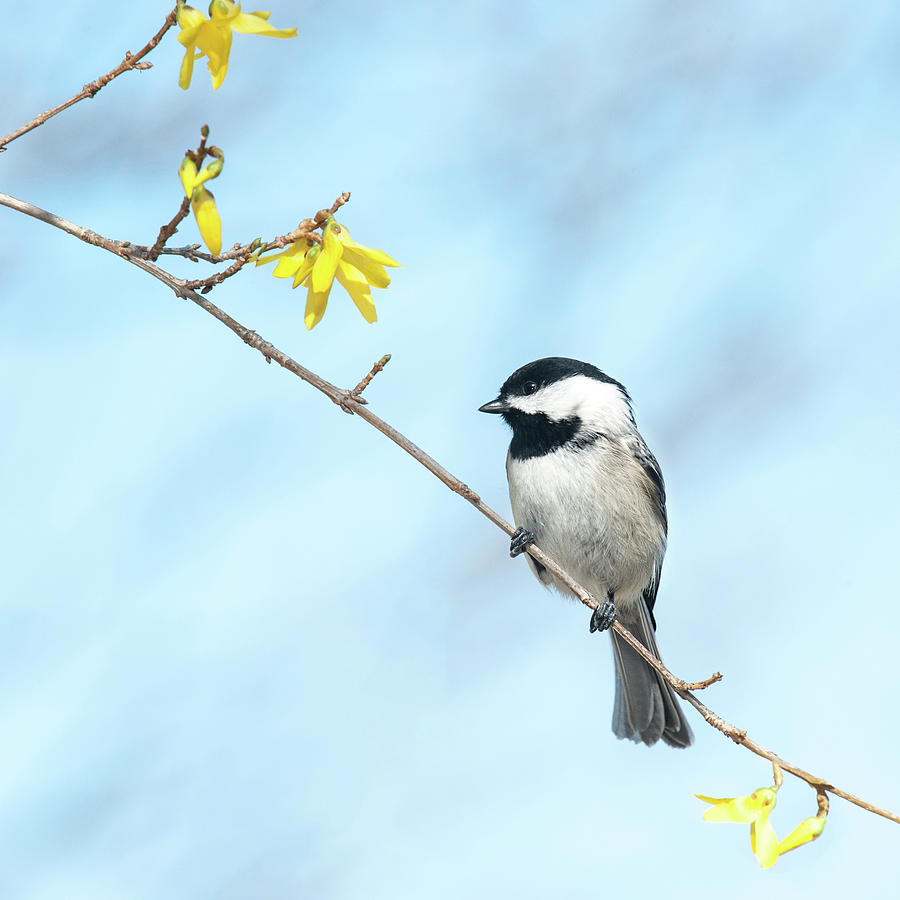In this detailed and photographic image set outdoors during the bright daytime, a small bird with a mostly white body, a gray tail, a black crown, and a very tiny but pointed beak sits in profile from right to left on a thin brown branch. The bird's head is inclined slightly toward the bottom left-hand corner, and its small black eye and dark-colored beak are clearly visible. Its little feet, which are black-gray in color, grasp the branch amidst a delicate display of five yellow flowers, all with petals mainly pointing downward. Some petals appear to be falling off. The background features a light blue sky with hints of grayish-white clouds, adding a serene and airy atmosphere to the scene. The overall foreground is sharp and detailed, clearly focusing on the bird and the branch, while the sky in the background remains slightly blurred.